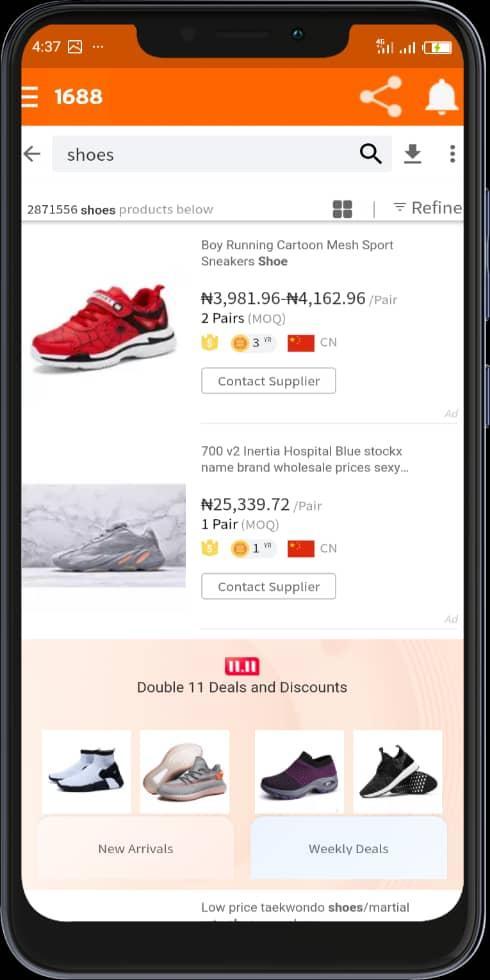The image is a screen capture from a mobile device, showcasing a shopping website with a white background and an orange trim at the top. The orange bar displays the time at 4:37 in the upper left corner. The main portion of the screen features a selection of sneakers, starting with a prominent display of a red sneaker on the left, characterized by a white and black heel detail. Beside the red sneaker, the price is listed, showing a range from 3,981.96 Naira to 1,062.96 Naira, with the Naira symbol denoted as an 'N' with two horizontal lines through it. Below the highlighted sneaker, an array of additional pairs of sneakers is also visible, suggesting a variety of options available for purchase on the website.